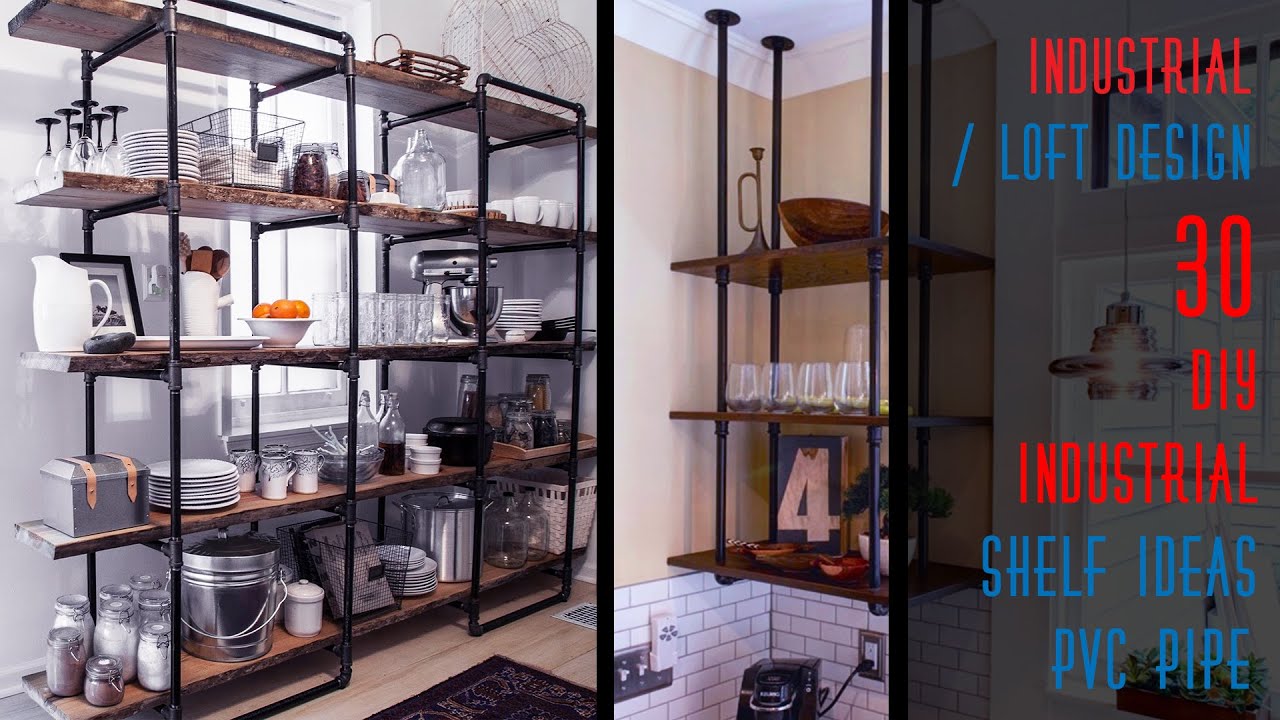The image is a horizontal, indoor color photograph of an elaborate shelving system that merges industrial and loft design elements. Dominating the left and center of the photo are tall shelves, constructed with sturdy metal pipes supporting thick, unfinished wooden planks, creating a raw yet stylish appearance. These shelves, totaling five tiers on the left and three in the center, are brimming with a variety of kitchenware, including plates, glasses, bowls, wine glasses, mason jars, pots, silverware, and small kitchen appliances like a mixer and a Keurig coffee maker.

On the leftmost shelving unit, detailed views show a potted plant at the bottom, followed by neatly arranged wine glasses on the second tier, and a distinct blue rectangle with a white number 4 on the third tier. The center shelves, suspended from the ceiling by black rods capped with flat cylindrical pieces, highlight an assortment of glasses, candles, and décor items, one of which looks like an overturned trumpet.

On the right side of the image, a different set of shelves appears superimposed, seemingly hanging from the ceiling. Superimposed over this section is a large, vertically oriented banner with bold, all-capital text: "INDUSTRIAL" in red, followed by a blue backslash and "LOFT DESIGN" in blue. Below this, in red, is "30 DIY INDUSTRIAL" and further down in blue, "SHELF IDEAS, PVC PIPE." This section appears to blend seamlessly with underlying images that include a basket of plants and potentially a chandelier, enhancing the rustic industrial ambiance of the scene.